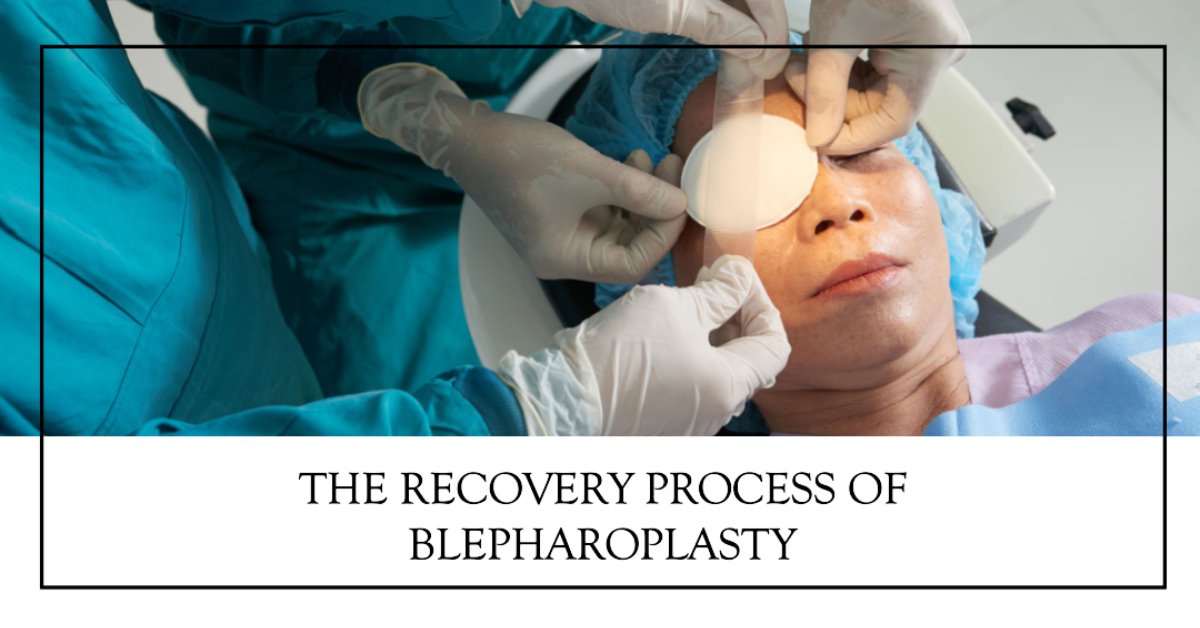This detailed image, resembling an ad or informational slide, depicts a woman's face being treated post-surgery, specifically from blepharoplasty. Four white-gloved hands, belonging to two surgeons clad in bluish-green attire, meticulously apply a circular gauze patch over the woman's right eye and secure it with tape. The woman, wearing a blue surgical cap and a purple gown, has pink lips and her face is framed by the surgeons' hands. The entire scene is encapsulated within a horizontal, rectangular black border, with parts of the surgeons' arms extending slightly beyond the confines of this border. Below the image, a white section with bold black text reads, "The recovery process of BLEPHAROPLASTY."